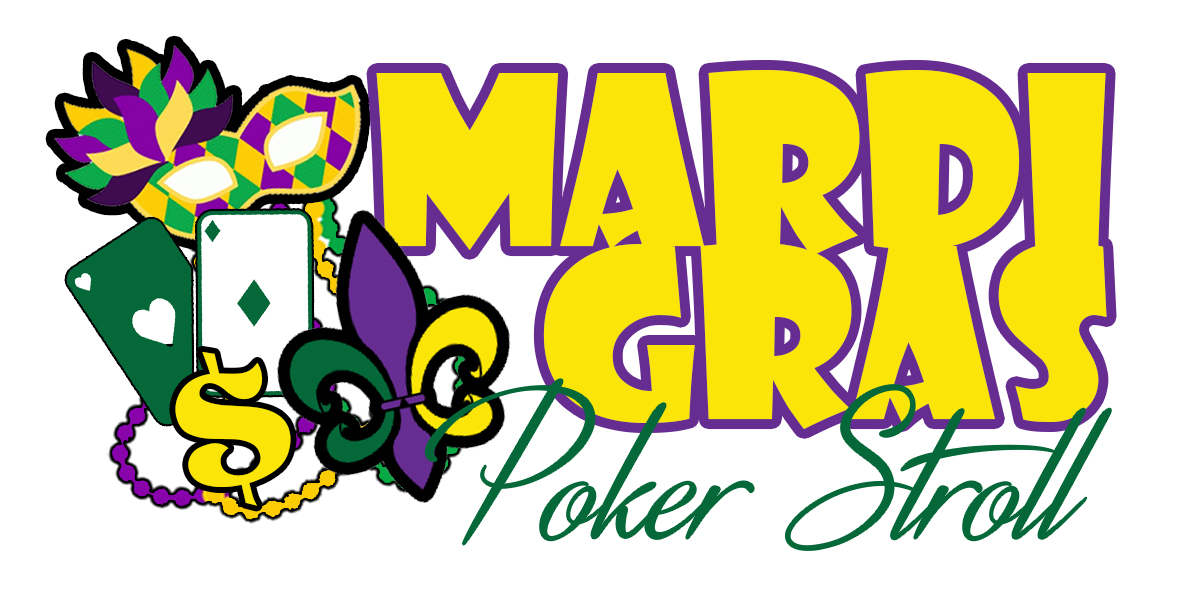The image is a vibrant, computerized advertisement for a "Mardi Gras Poker Stroll," featuring bold, eye-catching details. "Mardi Gras" is prominently displayed in large, bold, yellow sans-serif letters outlined in purple. Below, "Poker Stroll" is written in a smaller, cursive green font that slightly overlaps the main text. The image includes numerous Mardi Gras-themed symbols such as a green, purple, and yellow masquerade mask on the left, playing cards (a green heart on a white background and a green diamond on a white background), a yellow dollar sign, a string of purple and yellow beads, and the iconic fleur-de-lis in the traditional Mardi Gras colors of yellow, purple, and green. All elements seamlessly share the signature Mardi Gras palette, creating a festive and cohesive visual.